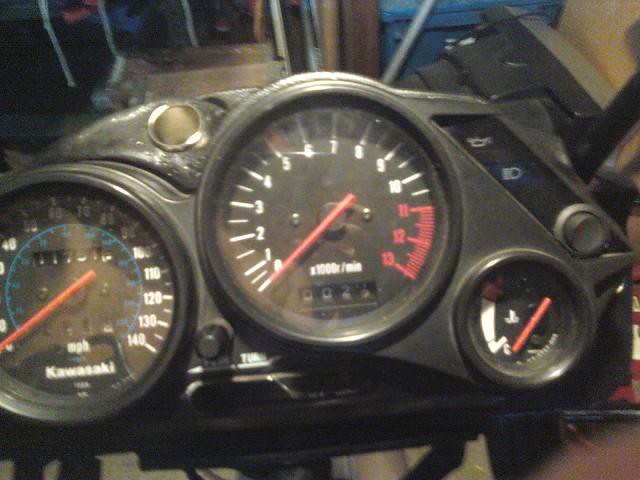This photograph captures the instrument cluster of a Kawasaki motorcycle. The panel features an older style with analog gauges: the speedometer on the left, which maxes out at 140 mph, and the tachometer centrally positioned, reaching up to 13,000 RPM. On the right, there is a temperature gauge that currently indicates the engine is cold. The odometer shows a total of 11,751 miles, hinting at considerable use.

The image reveals that the instrument cluster is somewhat dusty and dirty, with visible grime and smudge marks, indicating that this is not a brand-new motorcycle. The assorted wear and tear corroborate its history of use. Additionally, various indicator lights can be seen, including those for oil, bright and low headlight indicators.

The motorcycle is evidently parked undercover, as suggested by the muted, artificial lighting illuminating the scene. Overlaying this artificial glow, there is a faint hint of daylight at the top of the image, but it appears to be quite a dark day outside. This diffused light imbues the photograph with a slightly dim ambiance, emphasizing the weathered state of the instrument cluster.